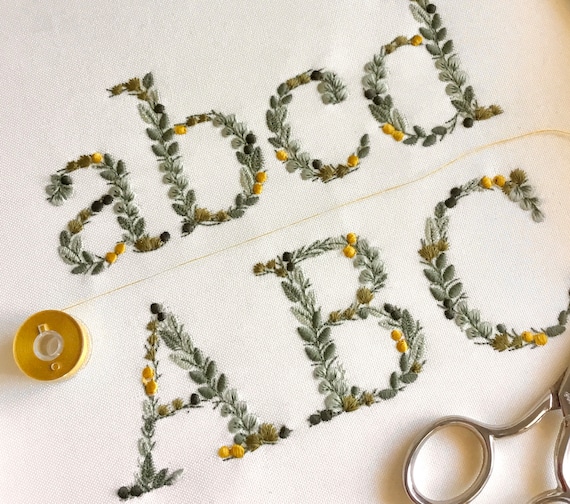The image showcases an intricate embroidery piece on an off-white fabric background. At the top, the letters "abcd" are meticulously stitched in lowercase, using various shades of green and yellow threads, giving them the appearance of being made from individual leaves and small flower buds. Below, a yellow spool of thread lies horizontally, with its thread pulled out to the side. Underneath the spool, the letters "ABC" are embroidered in uppercase, similarly crafted with leaf and bud motifs in light green, dark green, and yellow hues. In the bottom right corner, the tip of a silver pair of scissors is visible, completing the detailed scene of this creative sewing project.